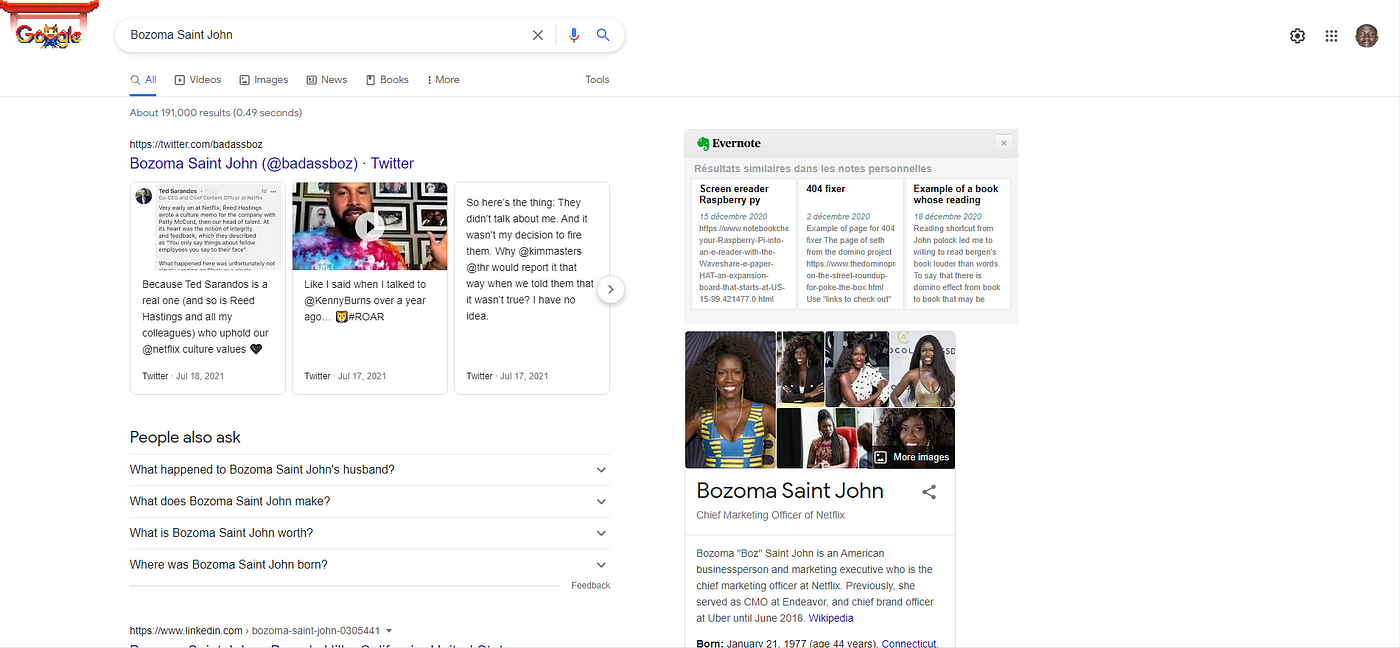The image appears to be a detailed screenshot of Google search results displayed on a desktop or laptop screen. The Google logo, located in the upper left corner, features a distinctive oriental theme, incorporating a red pagoda and a small cat in place of the second 'O'. The search query entered is "Bozoma St. John". Directly beneath the search bar, there are the standard navigation options labeled as "All," "Videos," "Images," "News," "Books," "More," with a "Tools" option to the far right.

The search has yielded approximately 191,000 results in a swift 0.49 seconds. The topmost result is a sponsored link to Bozoma St. John’s Twitter profile: https://twitter.com/badassboz. This result is presented with the title "Bozoma St. John (@badassboz) / Twitter" in blue text, accompanied by a visual layout of three side-by-side squares. The left square contains some textual information from Twitter, the middle square features an image which is a potential video thumbnail, and the right square includes additional information from the profile, though the small text is difficult to decipher.

Below the sponsored result, there is a section titled "People also ask" with four questions related to Bozoma St. John: "What happened to Bozoma St. John's husband?", "What does Bozoma St. John make?", "What is Bozoma St. John's net worth?", and "Where was Bozoma St. John from?".

On the right side of the search results, there is an information panel featuring Bozoma St. John. This panel seems to be associated with Evernote, displaying the green elephant logo and the text "Evernote" followed by some terms in another language: "resultats," "similarities," "done," and "les notes personales." Below this, there is additional English text mentioning "screen e-reader Raspberry Pi,” a label "404 fixer," and an example of a book being read.

The panel showcases six images of Bozoma St. John, illustrating her with different hairstyles including curly, bushy, and straight/wavy looks. The images collectively identify her as an African-American woman. Following the images, there is a segment from Wikipedia, identifying Bozoma St. John as the Chief Marketing Officer of Netflix. Although the small text is largely illegible, it confirms key personal details: she was born on January 21, 1977, making her 44 years old, and hailing from Connecticut.